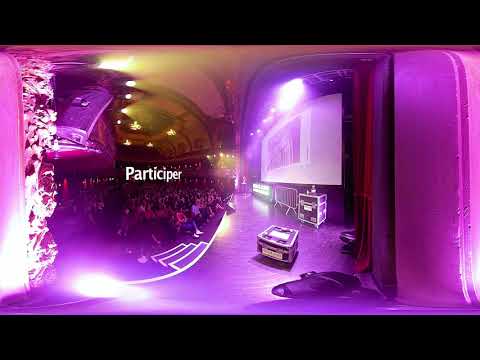Inside a room bathed in a purple hue, the scene is set with various lights and structures detailed throughout. White lights accent the environment, with a particularly bright one positioned at the bottom left corner and another to the far right. Central to the room is a bulge or circular shape featuring the white text "Participer." To the right of this text is a staircase leading down to a gathering of people.

A stage occupies the right side of the image, adorned with container boxes that could be for musical instruments, suggesting durability. A bright yellow light shines out from the top left corner across the ceiling, illuminating a large white screen at the top of the stage. This screen has a purple image with a white outline. 

On the left side, a textured, rocky column can be seen, possibly part of the wall, creating a unique visual element. At the top right, bright lights shine down on the stage, contributing to the vibrant ambiance. The atmosphere, augmented by a potential VR or 360 filter, contributes to a dynamic portrayal of a performance venue with an engaged audience looking on.